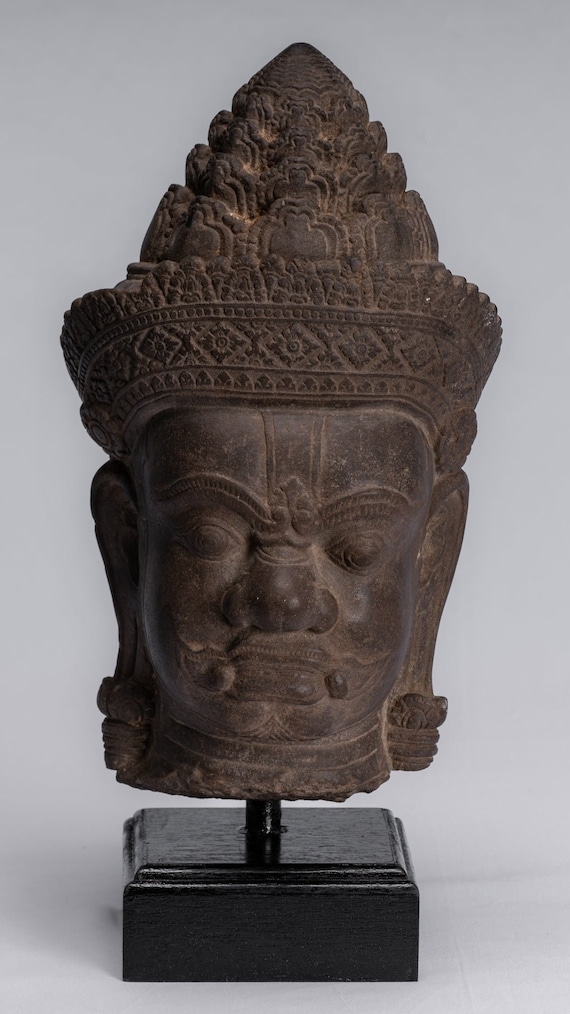This is a photograph of an intricate stone statue, most likely an idol or deity from Southeast Asia, perhaps Thailand. The dark sculpture, resembling bronze, depicts a head mounted on a black wooden base, connected by a short black rod. The face features a squat nose at the center, flanked by two prominent, slightly bulging eyes. Distinctive striped eyebrows slope downward towards the nose, adding a unique character to the visage. The lips are detailed with two small dots on either side, and the head is adorned with elongated ears, ringed near the lobes.

Above the face, a lavish, decorative headpiece crowns the statue. This ornate crown has a broad band embellished with a repeating diamond pattern around its center. Rising above this, the crown narrows into a pointy top, layered with a wavy, M-shaped tag pattern, culminating in a sharp, plain tip. The entire sculpture exudes a sense of ancient artistry and cultural significance, making it a captivating piece.